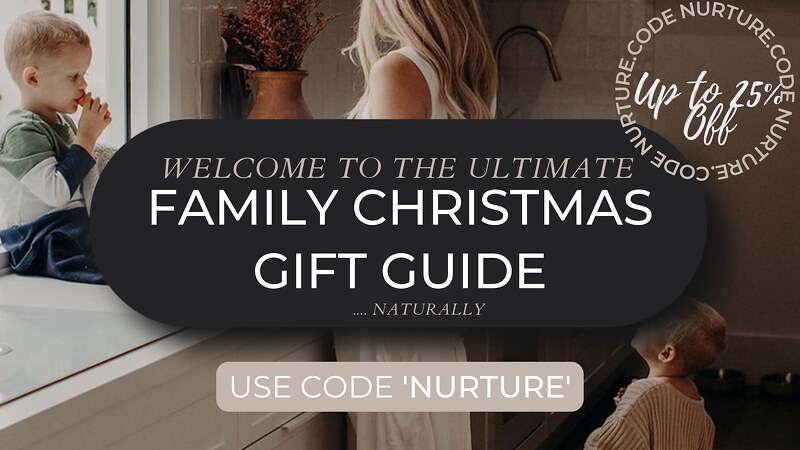In a cozy and inviting home setting, a mother in a long white dress gently leans against a white dresser, creating a scene of familial warmth. Her two young sons are with her—one, wearing a green and white shirt with jeans, sits comfortably on the counter, enjoying a snack, while the other, dressed in a peach shirt, stands close by, gazing up at his mom. In the background, a vase of fresh flowers adds a touch of nature to the homely environment, partially obscured by an advertising banner. The centerpiece of the image features bold white text on a black tag-shaped background that reads, "Welcome to the Ultimate Family Christmas Gift Guide, Naturally." An icon in the top right corner announces, "Up to 25% Off," and a circle nearby prominently displays the promo code "Nurture." Along the bottom, a gray box highlights the text, "Use Code 'Nurture.'" This heartwarming scene is designed to attract shoppers looking for the perfect gifts for their family this Christmas season.